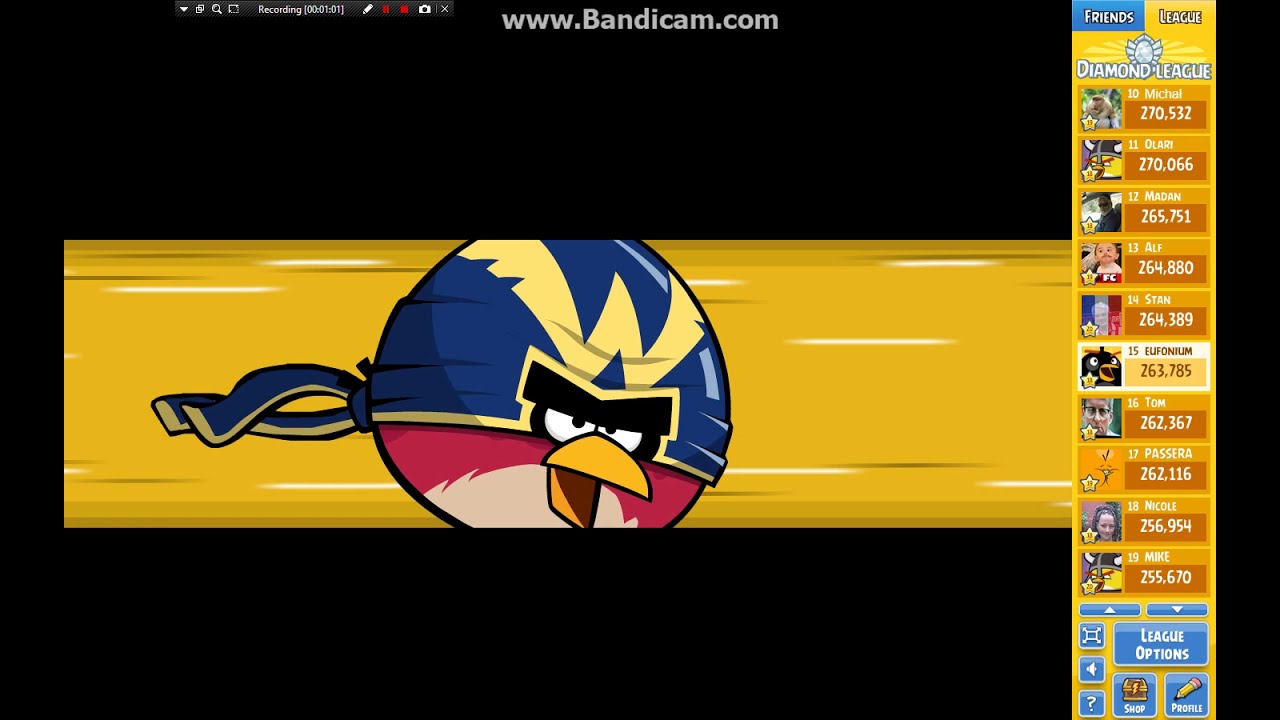The image is a screenshot, likely from the video game "Angry Birds," prominently featuring a cartoonish red bird character with a round face. The bird has a cream-colored underbelly and an expressive, furrowed brow, characteristic of the Angry Birds design, suggesting its angry demeanor. It is adorned with a blue and gold bandana, featuring a 'W' on its forehead. The bird appears to be flying to the right, towards the 3 o'clock direction. The background surrounding the image is a golden hue with white horizontal streaks, giving the scene an animated feel. The top of the image displays the URL www.bandicam.com, indicating the image is a screen recording, which has been active for one minute and one second. The top and bottom thirds of the image, as well as a small portion on the sides, are bordered by black bars. On the right-hand side, there's a vertical bar labeled "Friends" and "League," showing a leaderboard with multiple players' profile pictures and scores, suggesting a competitive element. Additional UI elements such as text in the upper left corner, a drop-down arrow, a magnifying glass, and some links in red are also visible.